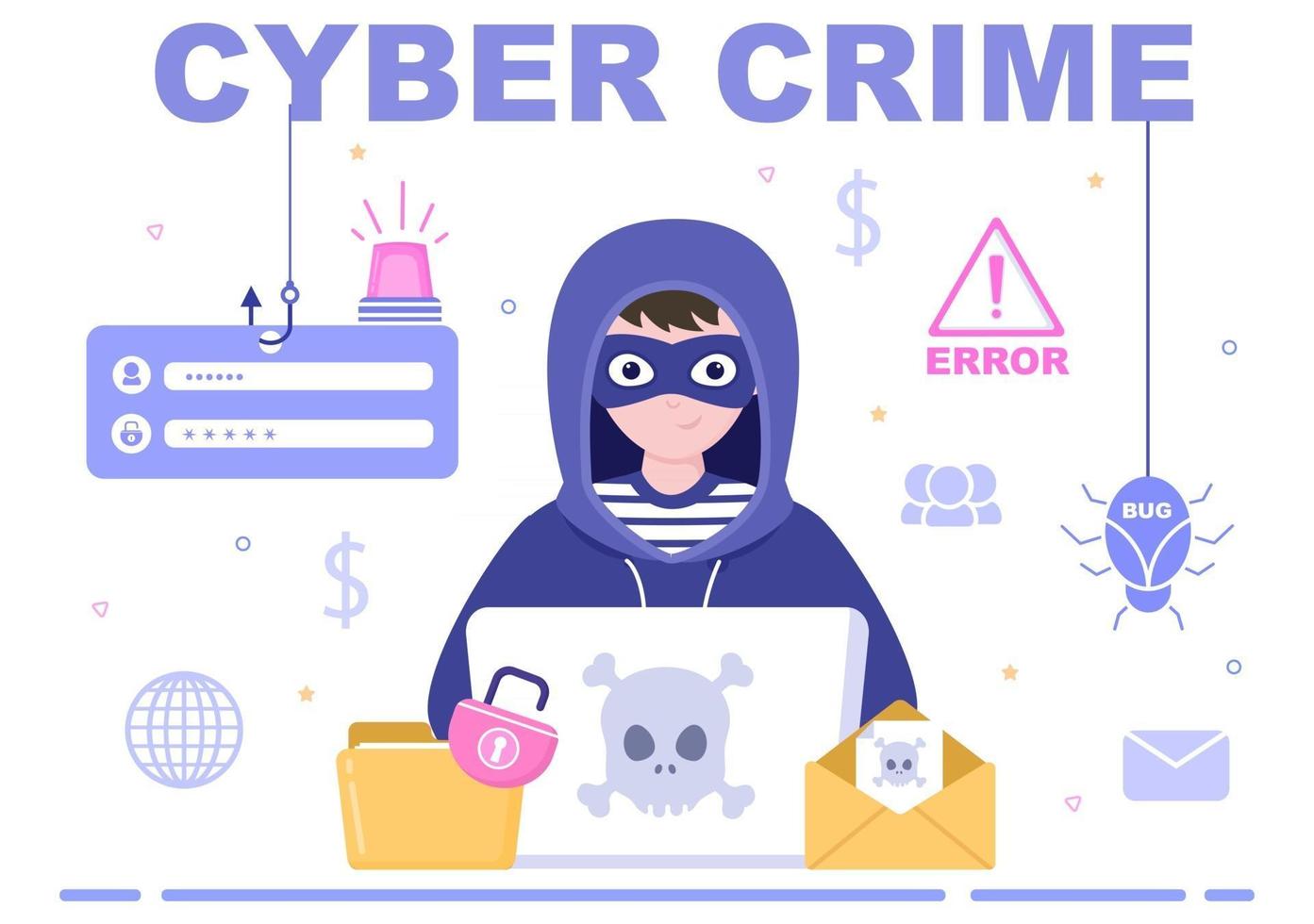The image is a detailed cartoon caricature with a light purple background, titled "CYBERCRIME" in bold, purple block letters at the top. Central to the image is a person depicted in a purplish-blue hoodie and a purple burglar mask, obscuring their face except for their brown bangs and eyes. They wear a purple and white striped shirt. The individual is focused on a laptop displaying a skull and crossbones on its screen. Surrounding them are several elements: to the left, a manila folder and a brown envelope, each containing a piece of paper with a skull and crossbones symbol. Additionally, a pink lock, a tan bin, and a purple rectangle with icons can be seen. A noticeable fish hook descends from the 'Y' in "CYBERCRIME," linked to an empty hook and a login information box, while a pale purple bug labeled "bug" hangs on the right. Nearby, a pink triangle with an exclamation mark signals an "ERROR." In the background, various symbols including dollar signs, a globe, and a group of people add to the theme of cybercrime.